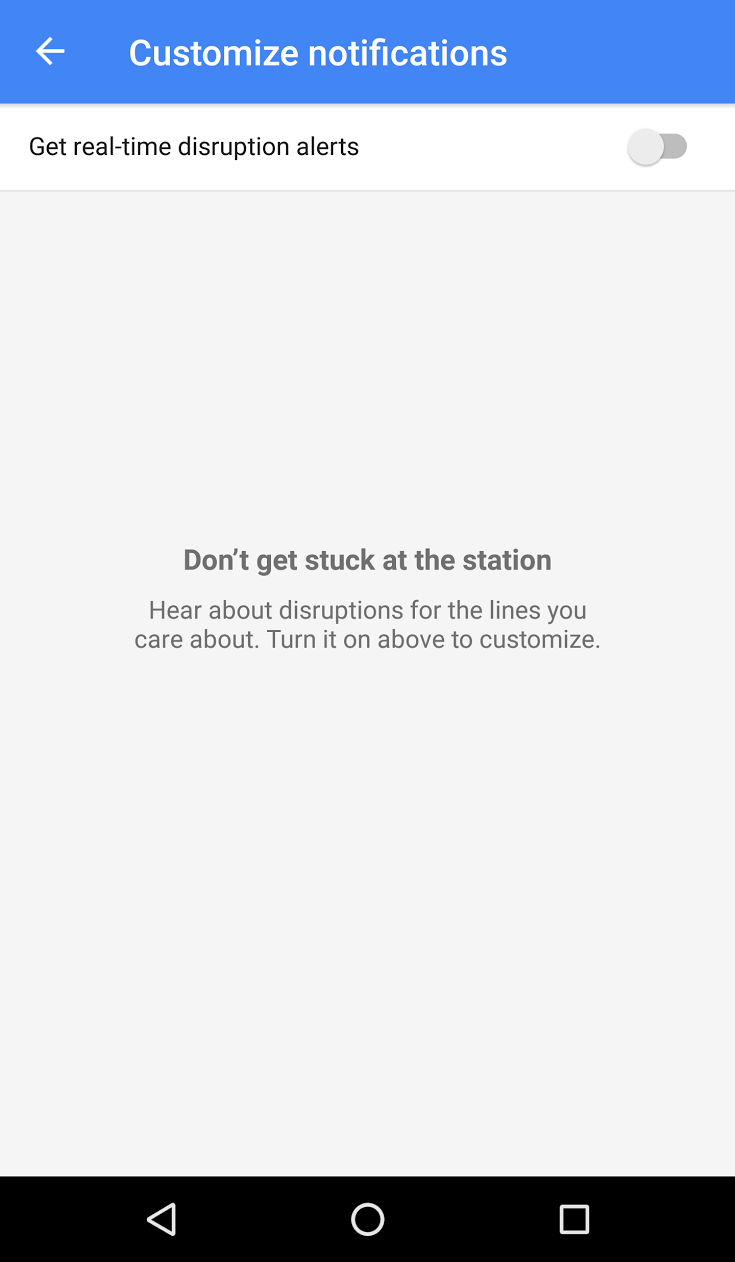The image features a light blue background. At the top, there is a bright blue box containing a left arrow icon and an option for customized notifications. Directly beneath this is a white box displaying the text "Get real-time disruption alerts" alongside a gray toggle switch. Below these elements, the light blue background includes a message: "Don't get stuck at the station. Hear about disruptions for the lines you care about. Turn it on above to customize." At the bottom of the image, a black box houses three symbols—a triangle, a circle, and a square—further emphasizing customization and alerts for real-time disruptions.